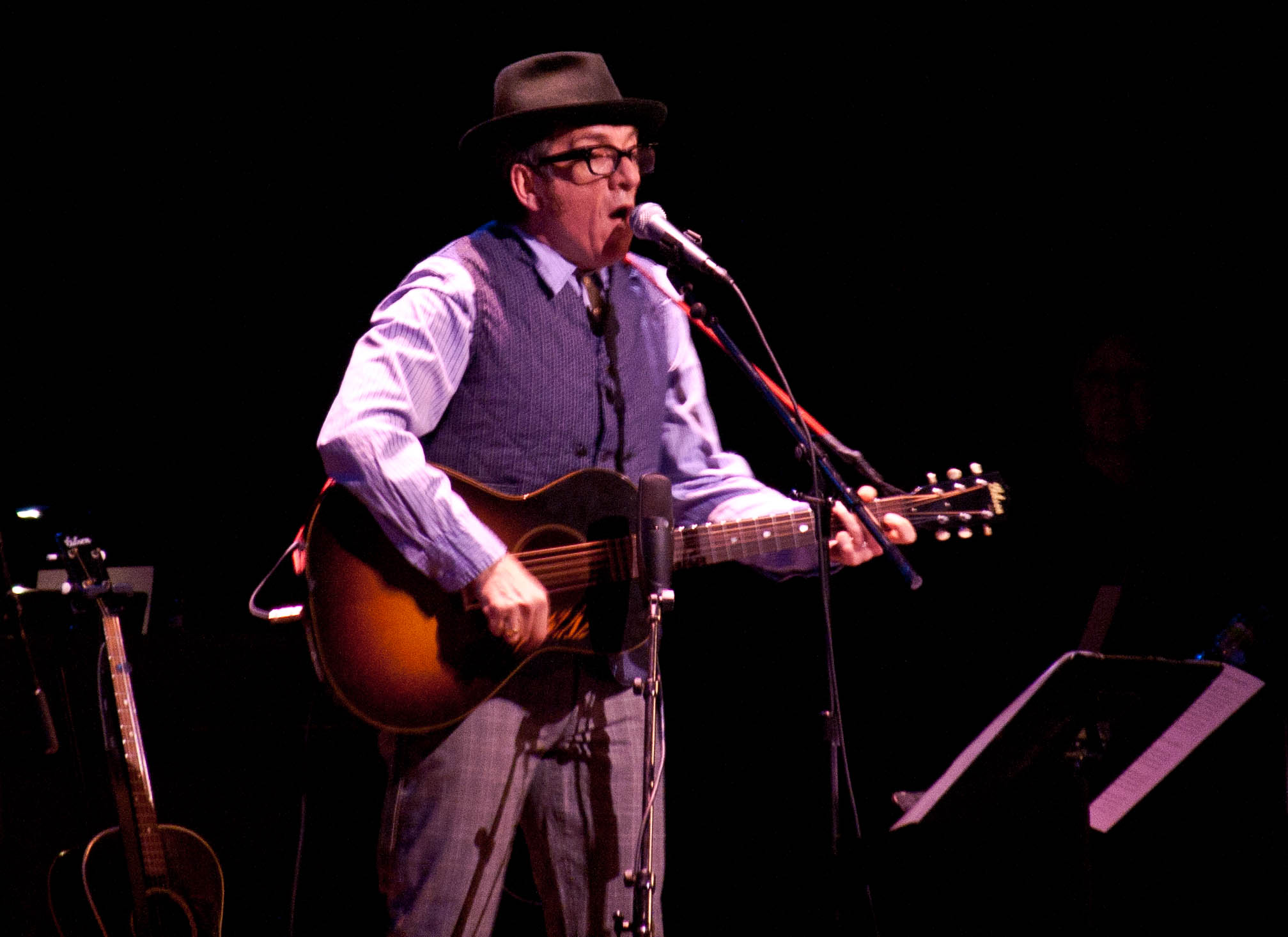A white male musician stands on a stage, passionately performing. He cradles an acoustic guitar, characterized by its wooden body stained in light and dark brown hues. The guitar is securely fastened with a strap over his shoulder while his hands are skillfully positioned, with one hand on the neck and the other near the base of the guitar. He sings into a microphone mounted on a stand in front of him. His attire stands out—a fedora hat and black-framed glasses, along with a long-sleeved t-shirt featuring white and blue stripes. Over the shirt, he sports a button-up vest, and he completes his outfit with grayish striped pants. The dimly lit background hints at additional musical equipment, adding to the atmospheric setting of the performance.